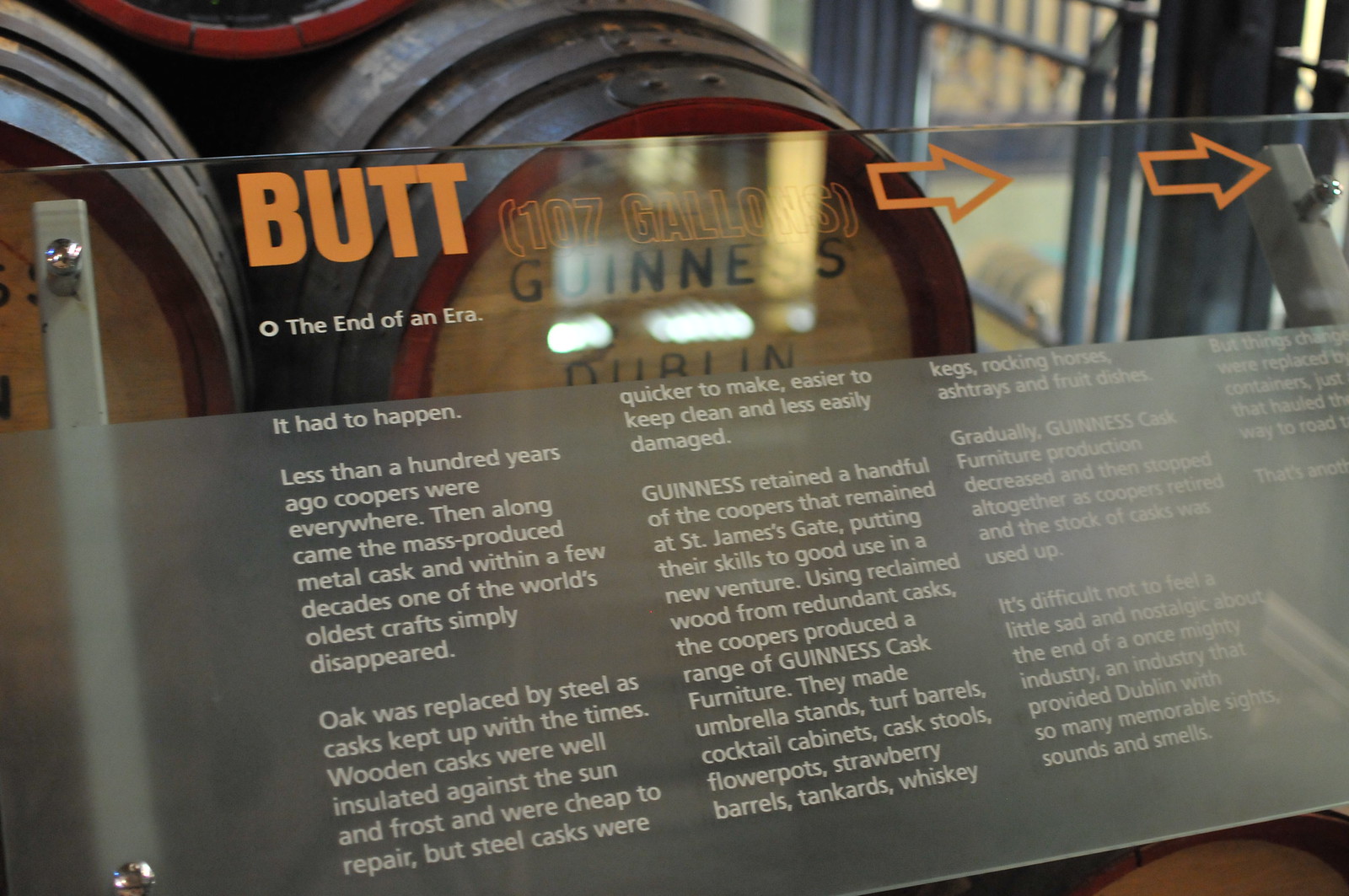The image depicts an informational plaque typically found next to a museum exhibit. The plaque appears to be made of clear and frosted glass, mounted on metal supports with visibility of casks in the background, notably one labeled "Guinness Dublin." The plaque's top section is clear with the word "BUTT" in orange capital letters, followed by "(107 gallons)" and two arrows pointing to the right. Below this, in white text, it reads "The end of an era." The main text starts with, "It had to happen. Less than a hundred years ago, coopers were everywhere. Then along came the mass-produced metal cask, and within a few decades, one of the world's oldest crafts simply disappeared." The narrative then details how oak casks, once insulated against sun and frost and cheap to repair, were replaced by steel casks, which were quicker to produce, easier to clean, and less prone to damage. The plaque continues, elaborating particularly on Guinness' transition to metal casks.